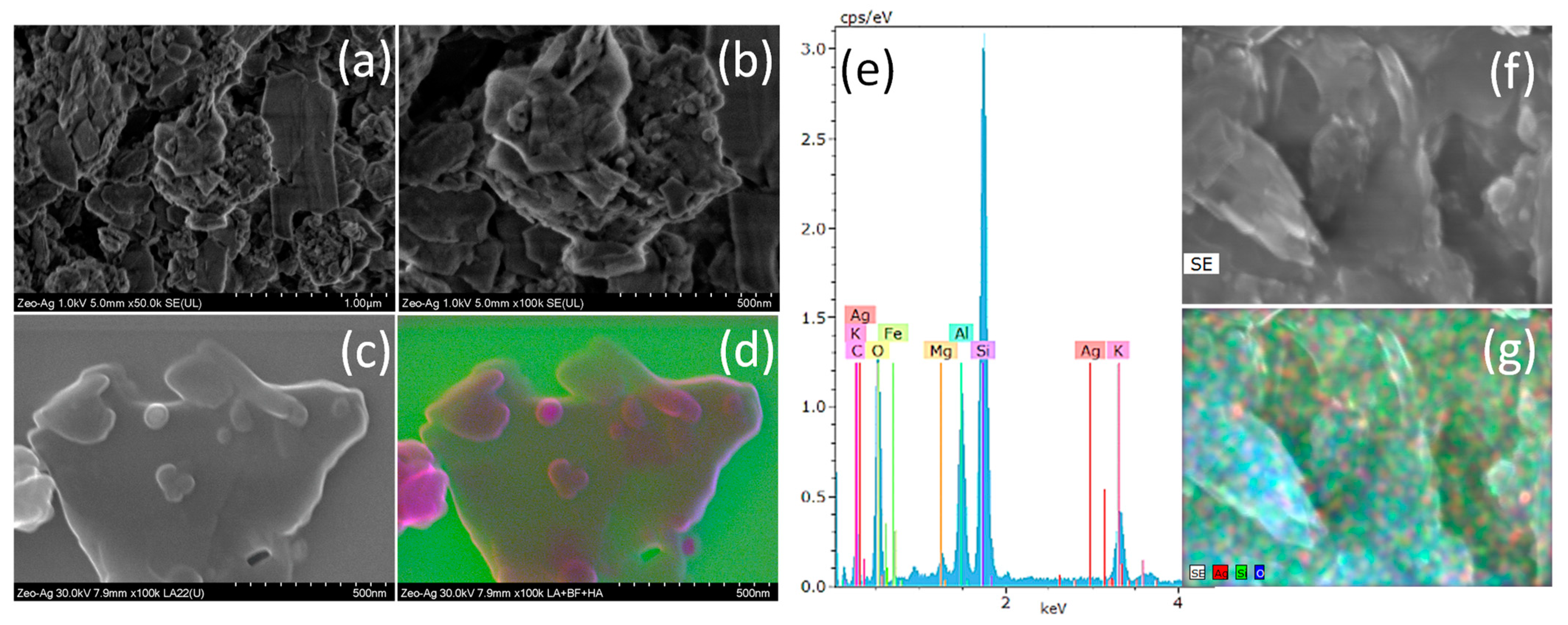The image showcases seven scientific visuals comprising a mix of detailed graphs and high-resolution microscope images. Labelled A to G, the visuals are organized with four on the left (A, B, C, D) and two on the right (F, G), enclosing a central graph (E). Images A and B in black and white display blurry, blob-like structures with distinct circular patterns, resembling microscopic organisms. Image C is also black and white, presenting a similar structure, while D, its colored counterpart, features vibrant highlights in hot pink and purple against a green backdrop. Images F and G, though appearing to depict crystalline rock formations, differ with F in black and white and G displaying a spectrum of rainbow colors. The central graph (E) aligns with the periodic table, showcasing chemical compositions with spikes on the y-axis labeled from 0 to 3, marked by colored lines in blue, pink, and red. Together, these images and graph appear to be part of a detailed scientific study, possibly exploring the intricate cellular or crystalline structures and their chemical compositions.